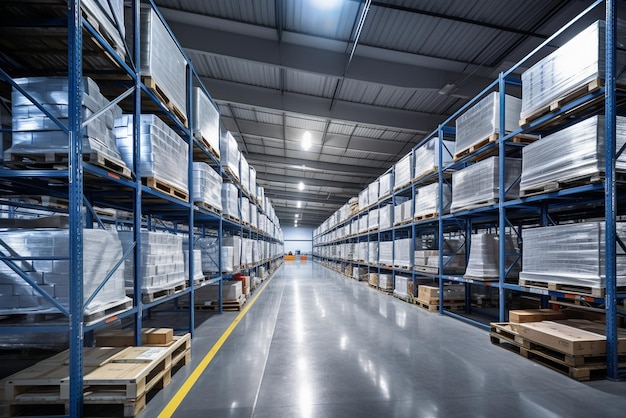The photograph captures a vast warehouse interior with an orderly arrangement of blue metal shelving units that stretch endlessly into the distance. Each shelf has four levels, stacked high with items wrapped in transparent plastic, most likely building materials such as cinder blocks. The shelves are organized into four rows, lining a broad, shiny concrete floor. Overhead, the metal ceiling features regularly spaced lights that illuminate the scene, casting a reflective glow on the polished surface below. A yellow line runs down the left side of the walkway, and in the far distance, indistinct shapes possibly represent two orange items and two people. The large gray metallic interior adds to the industrial ambiance of this expansive storage facility, which closely resembles those found in home improvement stores like Home Depot or Lowe’s.